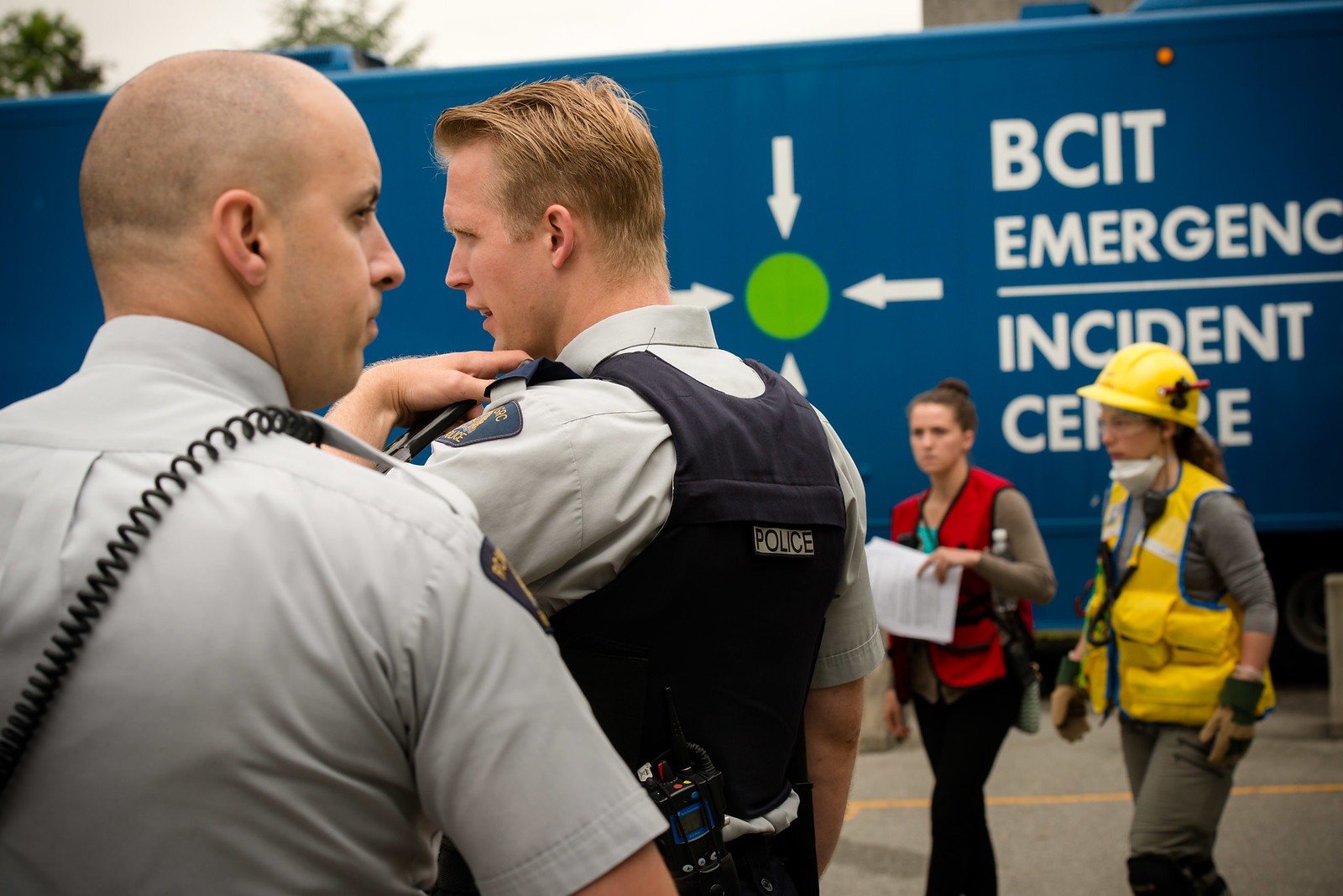In the foreground of this detailed image, an emergency scene unfolds with two police officers positioned on the left side. Both officers have their backs turned to the camera. The officer closest to the camera has a shaved head and is dressed in a light blue collared uniform shirt, marked with a blue badge on his shoulder that reads "POLICE". A black coiled wire is draped over his shoulder, and he gazes to the right. To his right stands another police officer with blond, combed-back hair, wearing a light blue uniform shirt under a blue padded vest that also displays "POLICE" on the back. This officer is speaking into a microphone attached to his shoulder.

On the right side of the image, there are two women, both engaged in what appears to be a coordinated response. The woman closest to the camera is clad in a yellow construction vest and a matching hard hat, equipped with a flashlight on the side. She also wears safety glasses and gloves. Next to her is a woman in a red vest holding a piece of paper. The backdrop features a street and a large blue trailer with "BCIT Emergency Incident Center" written in bold white letters, suggesting the scene is part of an emergency training exercise or a real incident in British Columbia. The trailer appears to be a mobile office used for staging, under an overcast, mid-day sky.